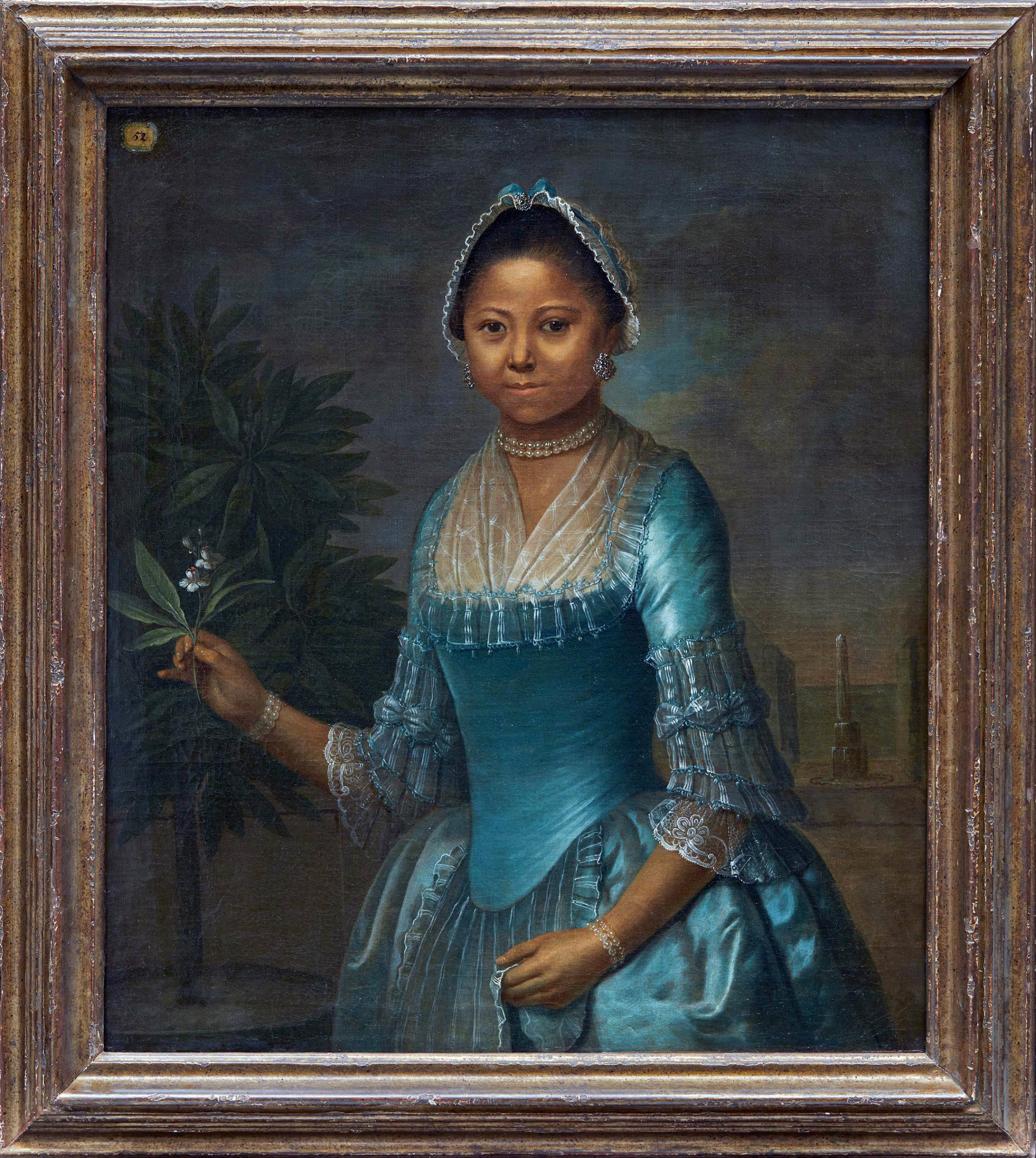The image is a detailed close-up of a hand-drawn painting of a small girl of African descent, characterized by her dark brown skin tone. The girl is depicted in a serene outdoor nighttime setting, captured in what appears to be an older, historical style reminiscent of the 1800s. She wears a light blue, ruffled nightdress with delicate frills at the ends of the sleeves and skirt, and a bonnet that conceals her black hair. Adorning her neck is a choker, possibly made of pearls, and small white ivory earrings dangle from her ears. 

Her right hand holds a fern or herb, while her left hand clasps a portion of her dress. The background highlights a large herbaceous tree, possibly a palm tree, and a statue or pylon structure that resembles a water fountain. The painting itself is framed with dark brown wood, and a small gold square mark is visible in the top left corner. The girl also wears lace-like bracelets on both wrists, adding to her historic attire. Her expression shows a faint, gentle smile as she poses amidst the detailed, natural backdrop.